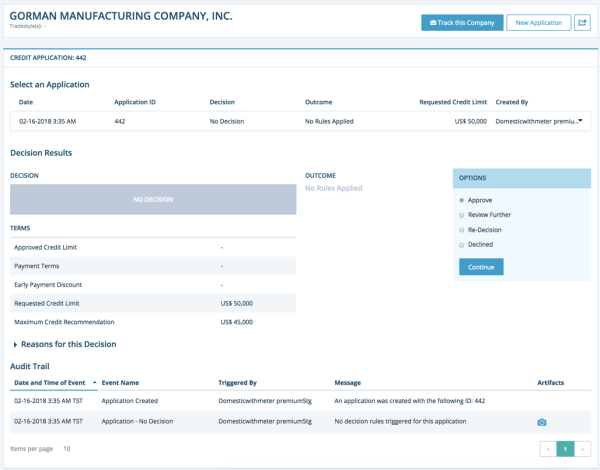The image displays a webpage from Gorman Manufacturing Company. The top of the page features "Gorman Manufacturing Company" written in light slate blue against a white banner background, which is set over a grey backdrop. To the right of this header, there are clickable options labeled "Track the Company" and "New Application." 

Below these options, there is a 3D cube displaying a smiley face graphic, though its purpose is unclear. The main body of the page pertains to a specific credit application, identified as "Credit Application 442." The application allows the user to select an application and displays a date of February 18, 2018, at 3:35 AM, along with the Application ID "442."

The current status of the application indicates no decision has been made, and no rules have been applied to determine an outcome. The requested credit limit is $50,000, yet the maximum credit recommendation is pegged at $45,000. Details about the application creator are provided, though specifics are not included in the summary.

Below, decision results state "No Decision" with a repeat mention of no rules being applied to outcomes. The user is given multiple options, including "Approve," "Review Further," "No Decision," and "Decline," with a button labeled "Continue" for submitting the decision.

Additional details reveal that no terms, approved credit limits, payment terms, quality payment discounts, or decision reasons are provided. The reasons for the decision involve some domestic issues with meter pre-funding, leading Gorman Manufacturing Company to decline this credit application.